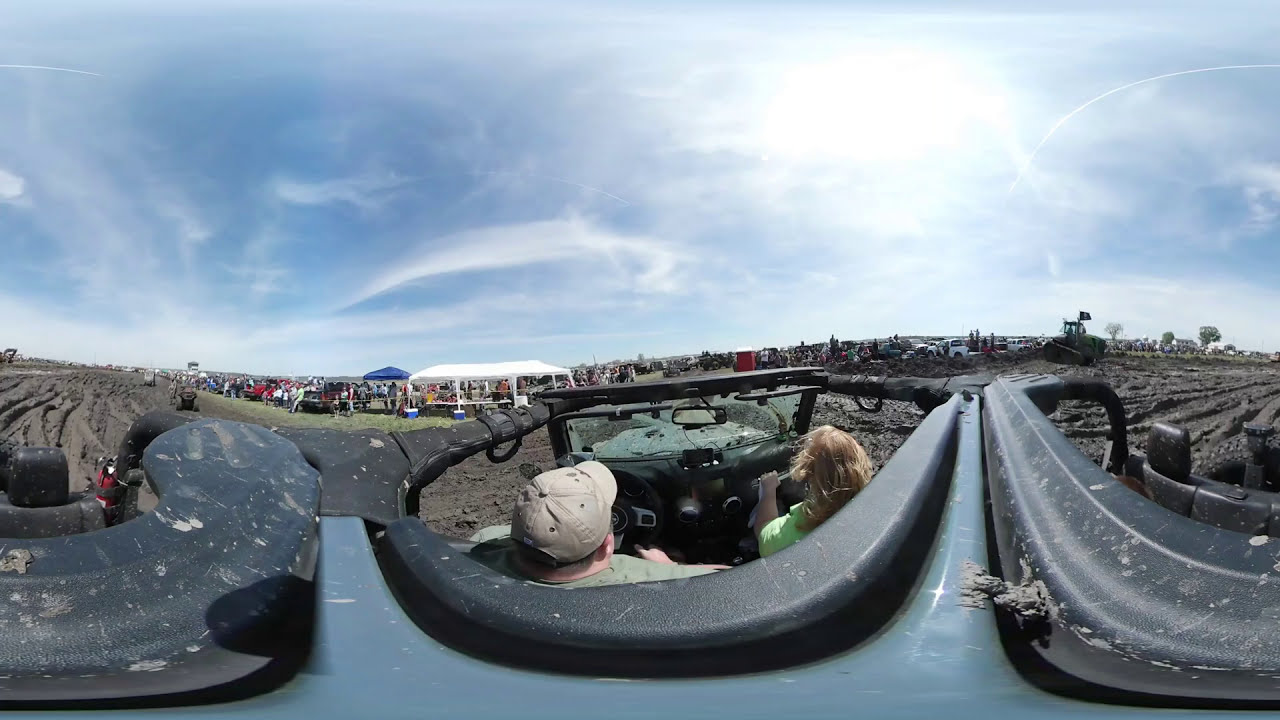The image, captured from a 360-degree camera mounted on the roof of an off-road vehicle—likely a jeep with a blue and black color scheme—shows a muddy terrain with prominent tire tracks. Inside the vehicle, a woman with blonde or reddish-orange hair, wearing a green shirt, is driving. A man wearing a beige or brown baseball cap sits beside her in the passenger seat. Both have their backs to the camera, making their faces unidentifiable. The scene ahead reveals a grassy area crowded with people and multiple canopies, with a notable white and blue top. Several cars are parked, and there is a large tractor with tracks and a flag on the right. The bright, sunny sky is mostly clear with some wispy clouds and a vivid sunspot visible. Behind the jeep, the muddy field stretches out, showing extensive tire marks and clumps of mud. Additionally, the jeep's interior includes a black dashboard with a screen and some leather seats visible.